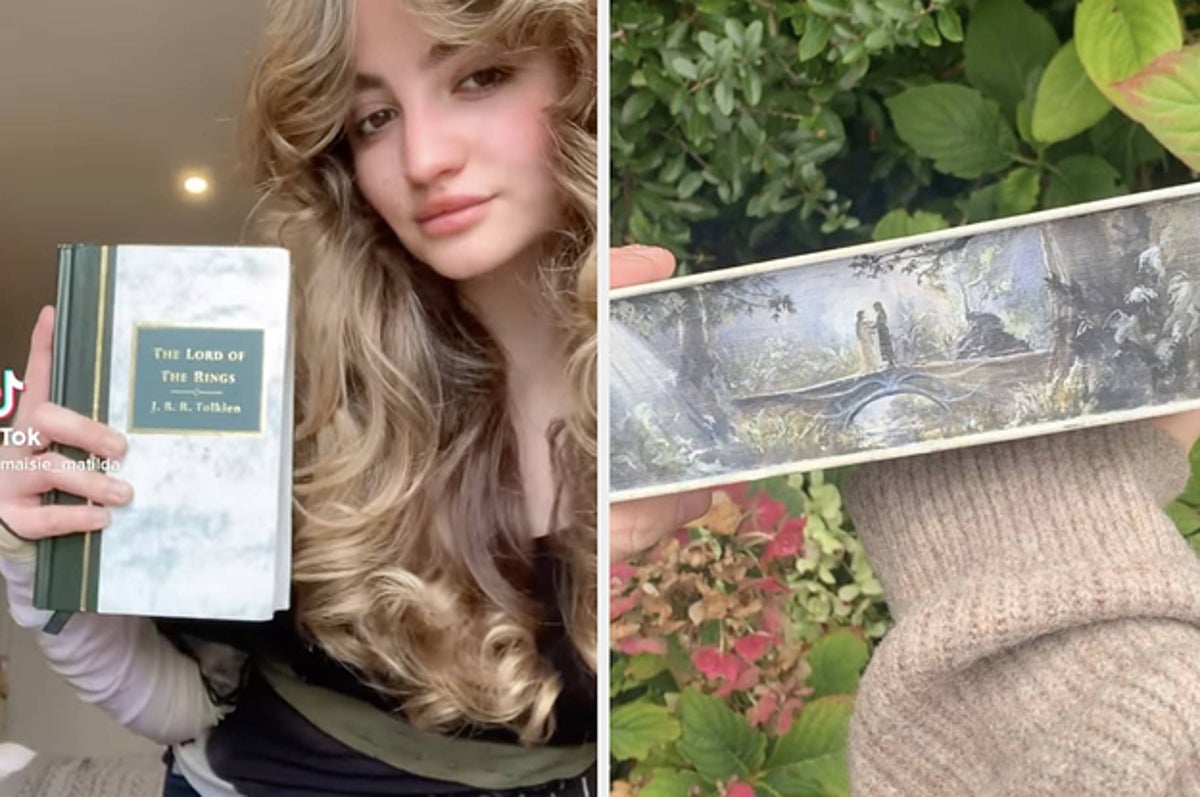This is a detailed full-color image divided into two sections. 

On the left side, there's a horizontal rectangle featuring a young Caucasian woman with long, flowy blonde hair. She is wearing a beige sweater which shows the emblem 'Tic Tac.' She is holding up a hardcover book titled "The Lord of the Rings," which has a white cover with a green rectangle displaying the title. The image seems like a screenshot from TikTok.

On the right side, the image is similarly horizontal and split diagonally. The upper part displays the woman's outstretched arm and her sleeve, while the lower part shows her hand holding a piece of paper, though partially obscured. Above these sections, leafy plants are visible in the background, indicating an outdoor setting. The piece of paper, resting on a corduroy sleeve, includes an old-style painting depicting a man and a woman standing on a bridge in an enchanted garden with a waterfall.